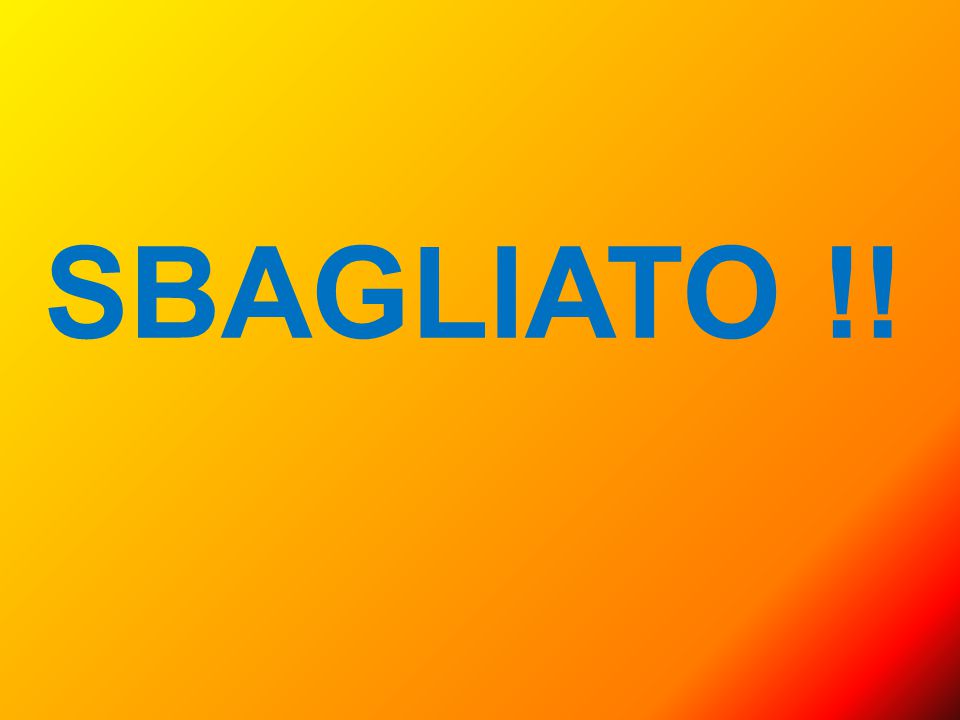The image features the word "SPAGLIATO!!" prominently displayed in dark blue, uppercase letters, slightly above the horizontal centerline of the frame. The vibrant background showcases a gradient that transitions smoothly from yellow in the top left corner, through hues of orange in the middle, to bright red in the lower right corner, and finally deepens into a dark red at the extreme bottom right. The colors blend seamlessly, with only a subtle, almost indistinguishable shift from yellow to orange, while the transition from vibrant red to deep red in the bottom right corner is more pronounced. There are no distinct objects in the image, and the overall style is reminiscent of a presentation slide, possibly created for a PowerPoint.